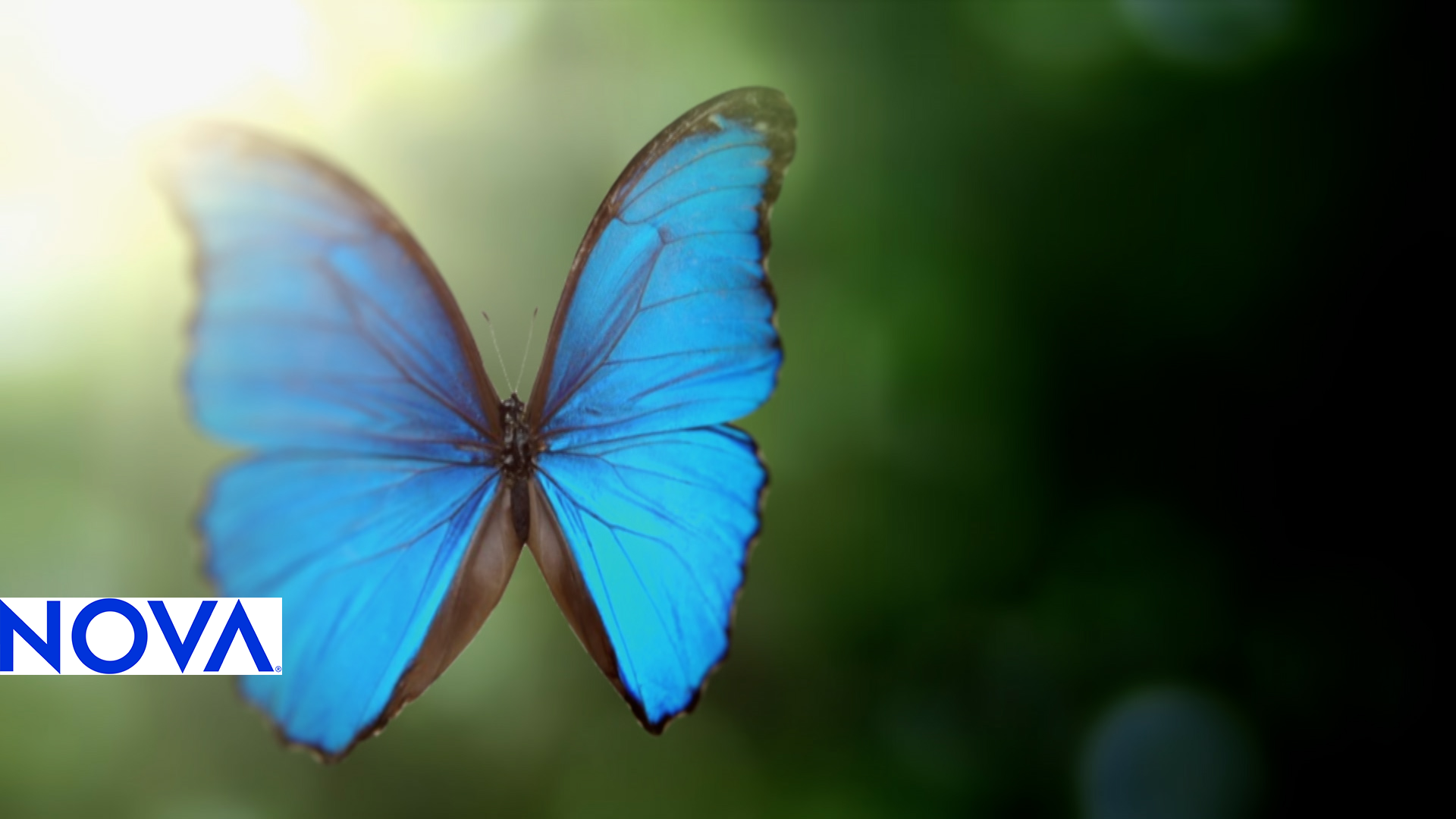The image, taken on a sunny day, features a striking turquoise butterfly with delicate, darker veins running through its luminescent blue wings and dark brown outlines. The butterfly appears to be in mid-flight with its wings outstretched and its black body, legs, and white antennae clearly visible. The background features a gradient of green hues, transitioning from a lighter mint color on the left to a darker shade on the right. A bright yellow sun illuminates the scene from the top left corner. In the lower left corner, there is a modern, minimalist white rectangle with the word "NOVA" written in blue letters; the letter 'A' in "NOVA" is notably missing its horizontal line. This butterfly is from the PBS show Nova, known for showcasing fascinating natural phenomena.